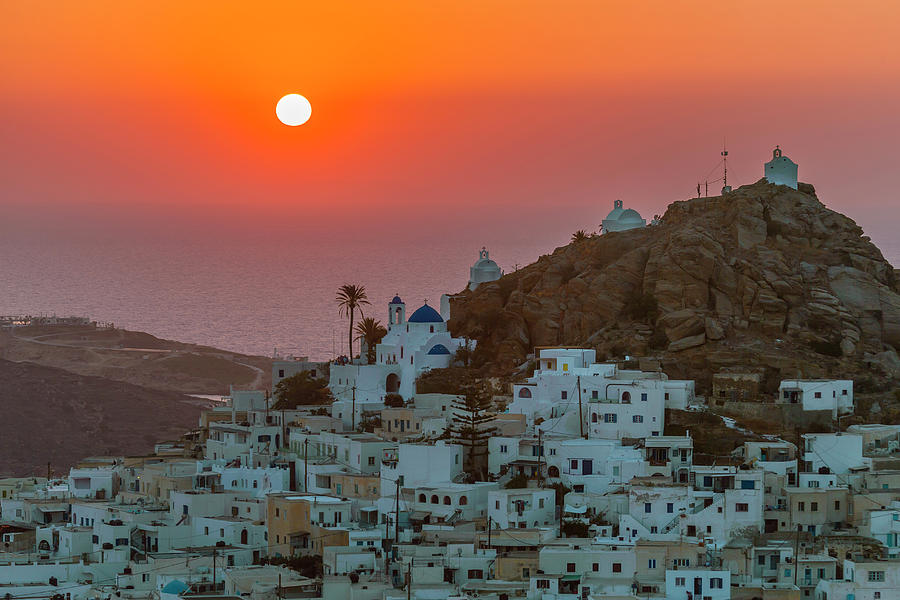This color photograph captures a breathtaking sunset over a whitewashed village built on a rocky cliffside. The sun, large and orange, sits low in a sky that transitions from deep purple at the bottom to a warm orange at the top. The calm water below mirrors these vibrant sunset hues, enhancing the serene atmosphere. The village comprises numerous small, square buildings with flat roofs, primarily concentrated at the base of the cliff, with a few climbing the rocky incline.

Clustered on the hill are several churches, the most significant halfway up the hill, distinguished by its white facade, blue roof, a small bell tower with an arched opening, and blue domes topped with crosses. Higher up the hill, three smaller white churches with bell towers stand prominently. The village's buildings, though mainly one-story, appear stacked like boxes as they ascend the cliff, featuring a mix of arched and square windows. Scattered among them are a few palm trees, adding to the picturesque scenery. Off to the left, the shoreline leads to a blue ocean stretching to the horizon, where the setting sun casts a warm glow over the tranquil landscape.